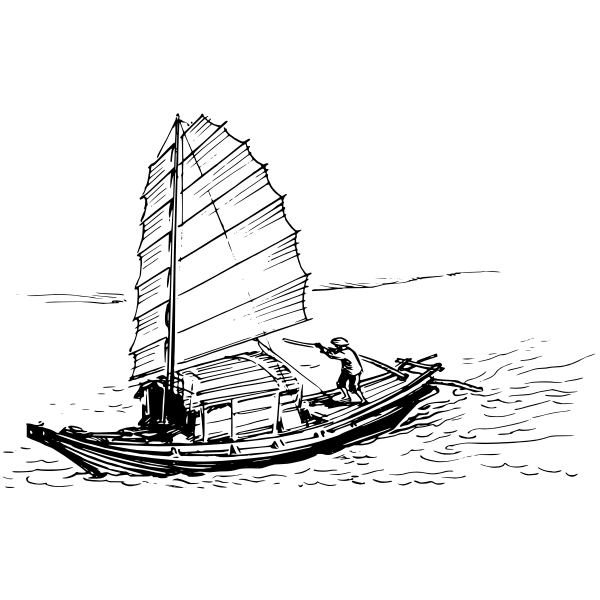The image features a black-and-white drawing of a sailboat centered on a solid white background, creating a stark and minimalist contrast. The sailboat, characterized by a rough sketch style reminiscent of marker or digital drawing, sits amid squiggly lines that represent water, adding a sense of movement and texture to the scene. On the boat, a single person stands, holding a large pole or paddle, though the lack of detail leaves the exact function ambiguous. The boat has a prominent single sail and a raised cabin area, suggesting a place one could go inside or below deck. The water appears calm, evidenced by the smooth background and subtle ripples around the boat, capturing a serene moment in the open ocean. The overall simplicity and monochromatic palette of the image evoke the feel of a coloring book illustration.